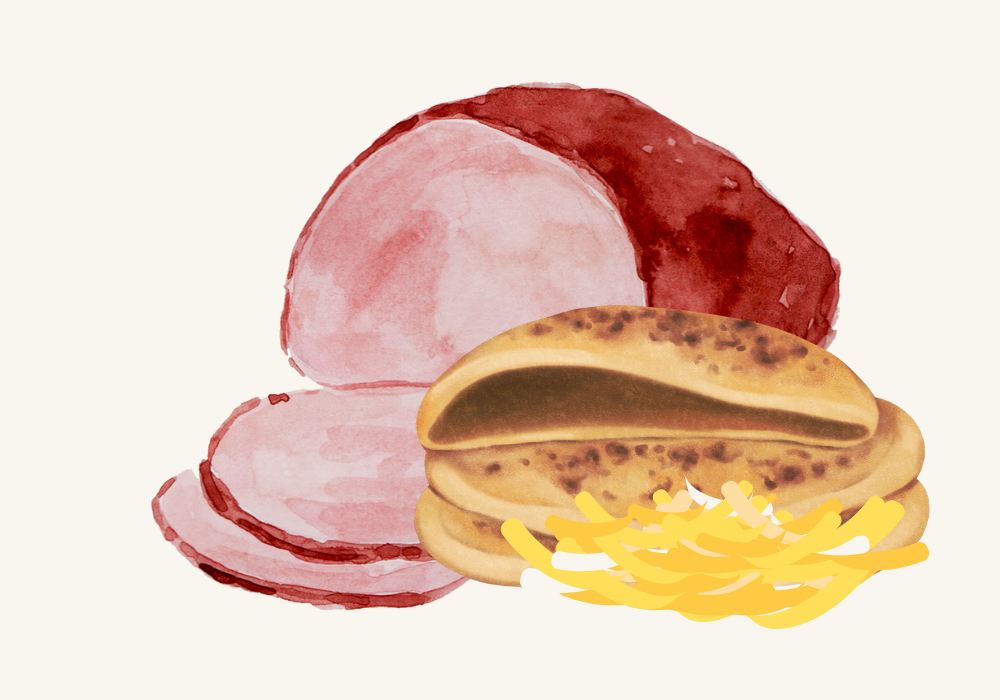This is a watercolor-style painting of a sliced ham and accompanying food items. The setting appears to be indoors, with an off-white or cream background. Central to the image is a piece of ham featuring a red outer surface and pink interior, sliced to reveal two pieces laid flat. Adjacent to the ham are three sections of what seem to be pita bread or soft taco shells; the top section is cut in half, showcasing its blackened, charred top and dark brown interior, while the two whole circular sections underneath are a matching light brown with some darker speckles. In front of the pita bread, there is a scattering of thin, yellow, and orange streaks resembling either french fries or shredded cheese. This detailed composition lacks any text, allowing the viewer to focus on the intriguing interplay of colors and textures.